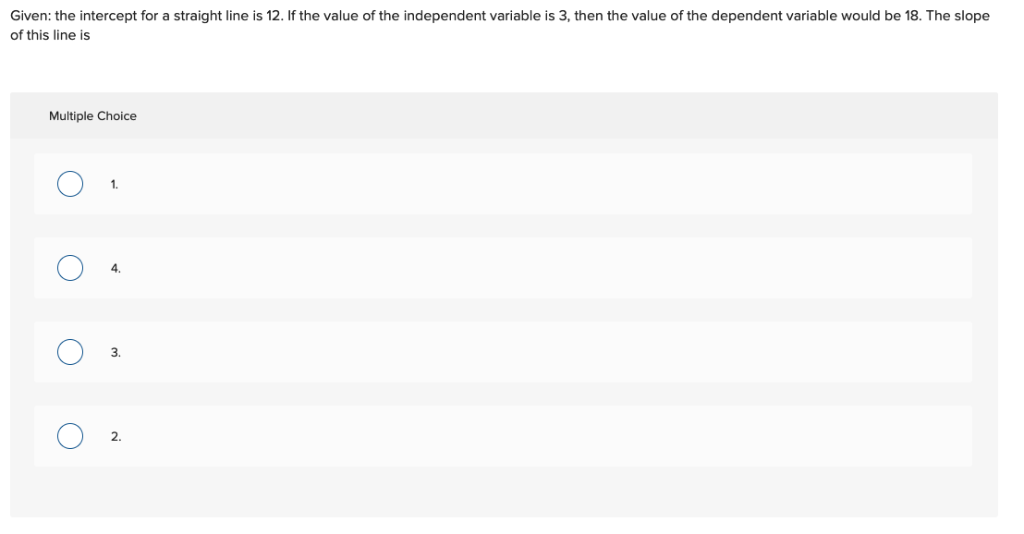Here we see a screenshot featuring a white background. At the very top, there's a black text that reads: "Given: The intercept for a straight line is 12. If the value of the independent variable is 3, then the value of the dependent variable would be 18. The slope of this line is." 

Below this text, there's a wide, light gray rectangle. In the top left corner of this rectangle, it says "Multiple Choice." Beneath this header, there are four lighter gray rows, each containing a white circle with a blue border to the left. These circles are numbered 1, 4, 3, and 2 respectively and indicate the selectable options for the multiple-choice questions. Interestingly, the numbers are not in ascending order, perhaps to emphasize the values being considered.

It seems this screenshot is part of an online quiz or test, where users must select one of the multiple-choice answers before moving on to the next question. The initial black text, due to its length, spans two rows, with "of this line is" starting on the second line.